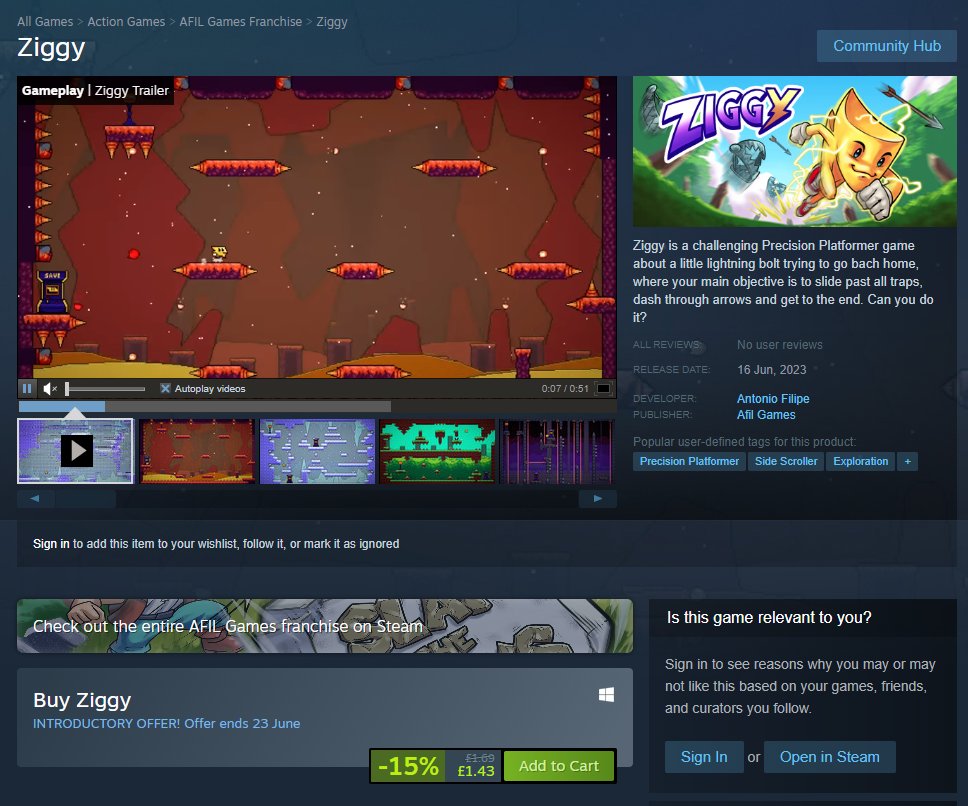The image depicts a Steam store page for the game "Ziggy." Positioned at the top left is the game's title, "Ziggy." Centered in the image is a representative screenshot from the game, showcasing its vibrant and dynamic visuals. "Ziggy" appears to be a precision platformer, featuring gameplay that revolves around a character who must skillfully navigate through various obstacles and traps. To the right of the image is a detailed description: "Ziggy is a challenging precision platformer about a little lightning bolt trying to go back home. Your main objective is to slide past all traps, dash through arrows, and get to the end. Can you do it?" At the bottom left, there's a call-to-action button that says "Buy Ziggy," with an attached note mentioning an introductory offer available until June 23rd for $1.43.